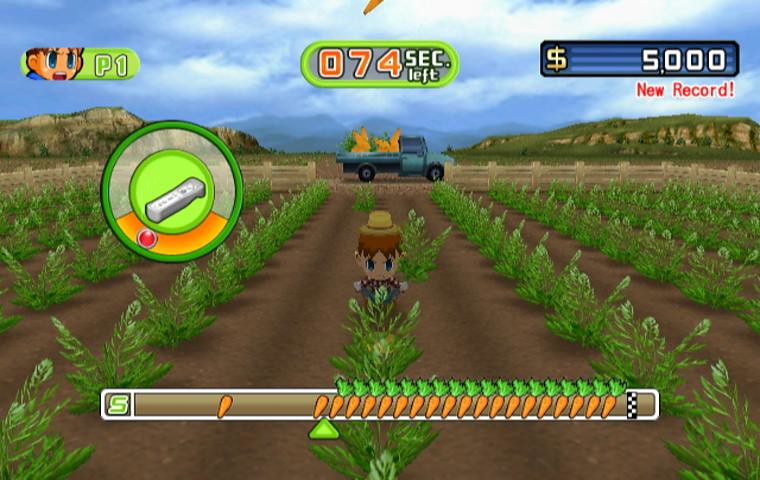This is a screenshot from a Wii farming game, depicted in a cartoony style. The main character, a young boy with brown hair and blue eyes, wearing a plaid shirt and a yellow hat, stands in the middle of a field of dirt rows with green plants, likely carrots. He is looking directly at the player. To the right of him, you can see a truck loaded with stacks of yellow and orange crops, behind a brown fence line. In the background, there are gray and brown rock hills under a cloudy blue sky. The top left corner shows "Player 1" with an avatar of the boy, and the top middle of the screen reads "74 seconds left." In the top right corner, the screen proudly displays "$5,000 new record." At the bottom, there's a meter filled with carrot icons indicating the collected carrots and a circular indicator featuring a white Wii remote.